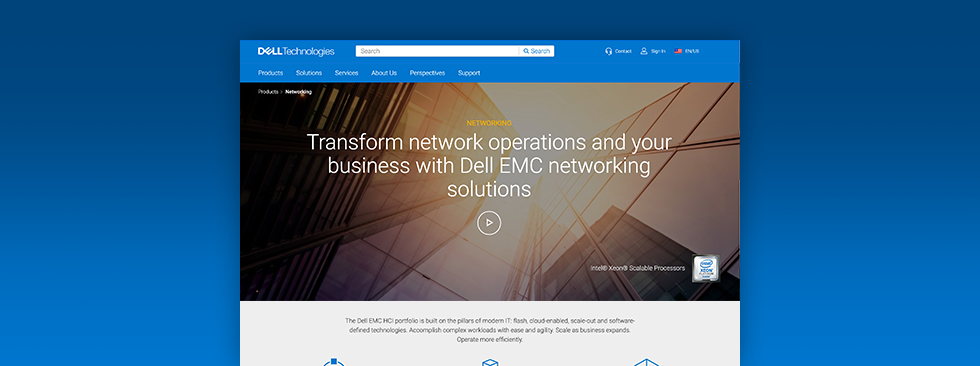The image features a rectangular design with a gradient blue background that transitions from a darker blue at the top to a lighter blue at the bottom. At the center of the image, there is a notable section displaying the text "Dell Technologies." Above this, a slightly discernible search bar is depicted along with a sign-in icon and several other functional icons.

Below the central part, various navigation options are presented, including "Products", "Solutions", and an "About Us" section. Additionally, there are two white sub-menu titles — "Transform Network Operations" and "Your Business with Dell EMC Networking Solutions," accompanied by a play button suggesting media content. Adjacent to the play button, an icon is visible on the right side.

The lower portion of the image transitions to a white background containing a centered paragraph. The very bottom edge includes the tops of several more icons, though they are partially obscured.